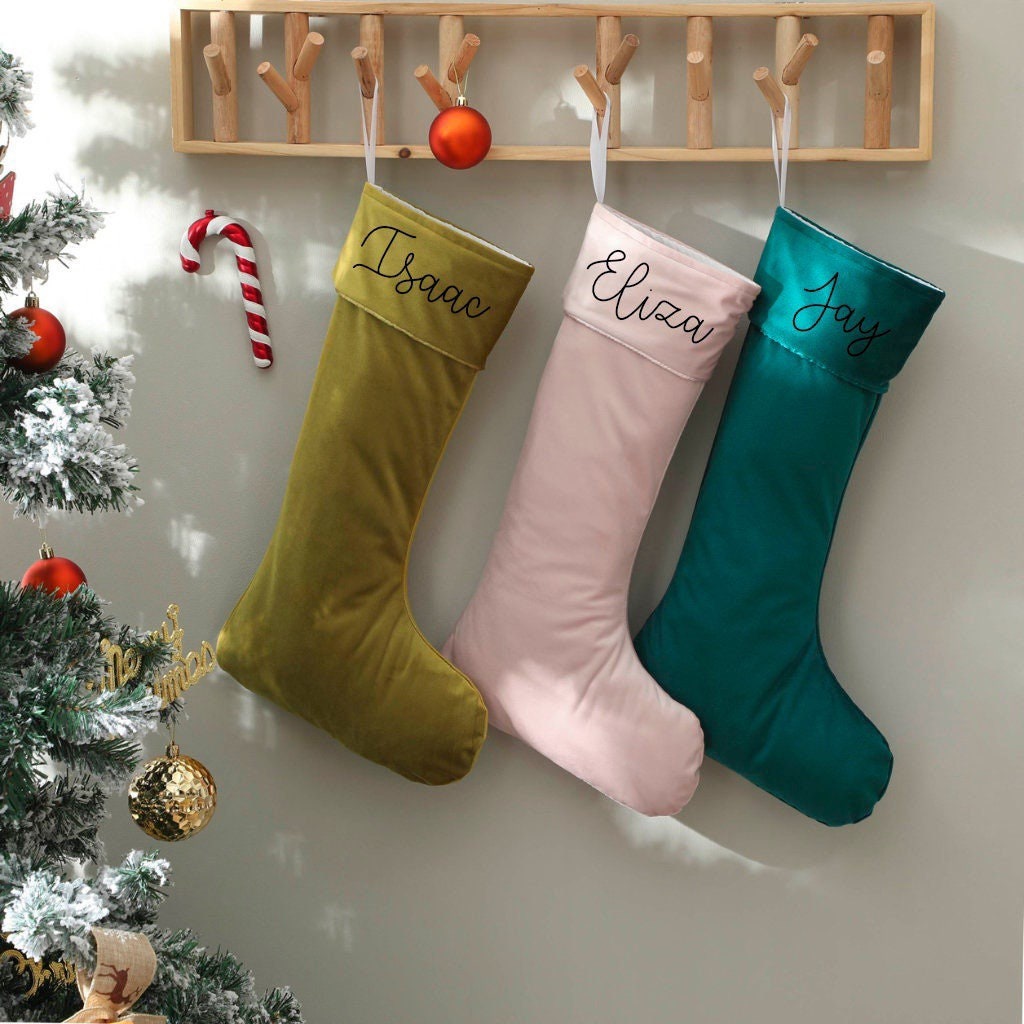This photograph, taken during the daytime, captures a festive Christmas scene. On the left side, a Christmas tree is adorned with green and gold baubles, brownish ribbon, and a gold sign that reads "Merry Christmas." The tree's dark green branches are dusted with fake snow. The focal point of the image is a wooden stocking holder designed to resemble branches set in a solid wood base. Hanging from this holder are three velvety stockings in bright colors: an olive green stocking embroidered with the name Isaac, a pastel pink stocking with the name Eliza, and a vibrant peacock teal stocking bearing the name Jay, all in a black cursive font. Additional festive details include a red ornament and a candy cane ornament hanging from the wooden holder. Sunlight illuminates the cheerful display, highlighting the softness of the stockings and enhancing the festive atmosphere.